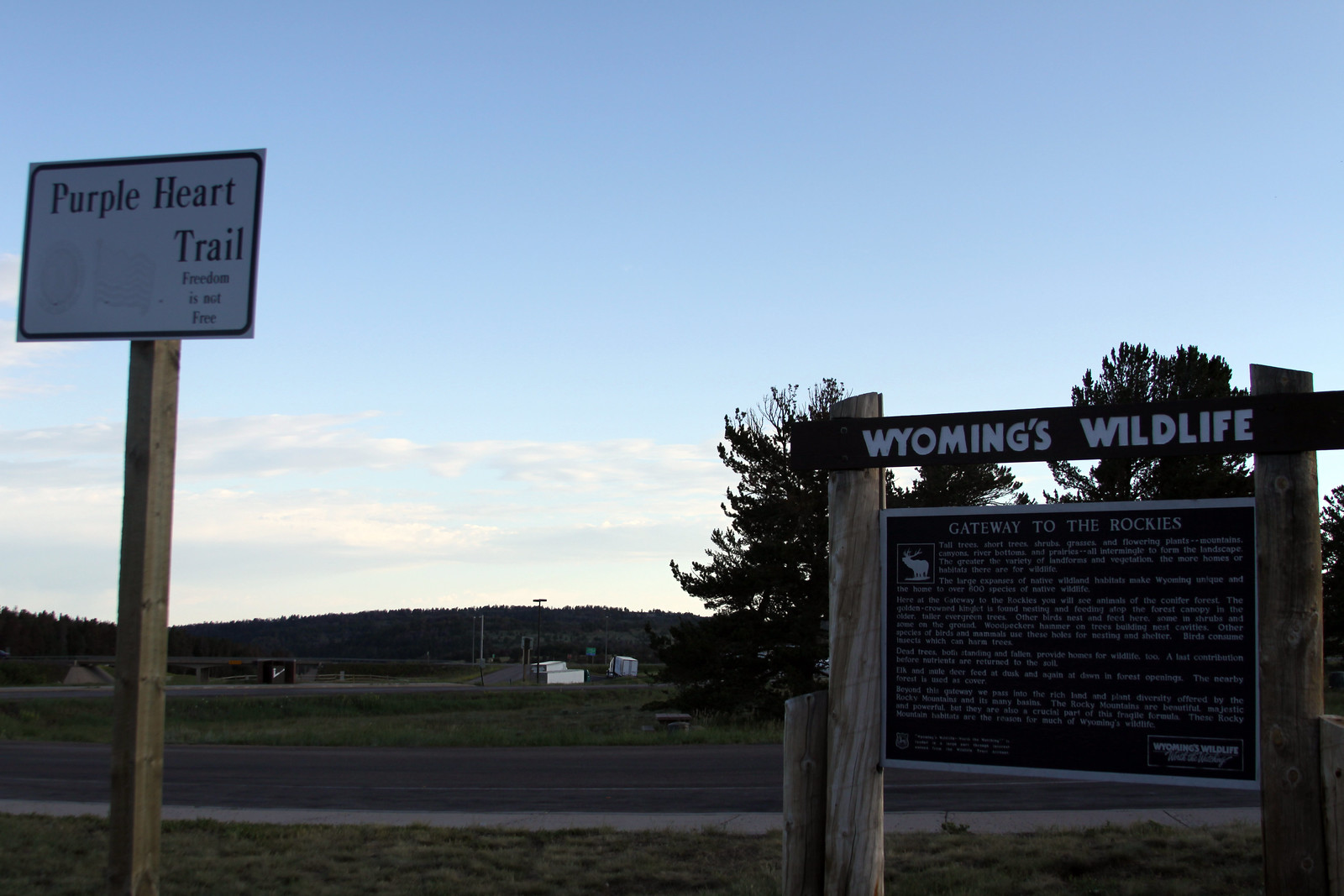The image captures a largely natural setting, likely taken outdoors during either dusk or dawn. The foreground features a grassy field crisscrossed by a highway. Just off-center to the left stands a wooden signpost displaying a white sign with a black border, containing black text that reads "Purple Heart Trail. Freedom is not free." Dominating the right side, a more prominent entry sign for "Wyoming's Wildlife" is visible. This larger sign is supported by two robust wooden pylons and has a plank of wood across the top with bold, white lettering that proclaims "Wyoming's Wildlife." Below, in a square-shaped section, it states "Gateway to the Rockies" alongside an image of a moose or elk and several paragraphs of text. The sky, sporting a blend of light blue, white, and gray hues, hovers above sparse clouds, suggesting the time as either early morning or late evening. In the background, a few houses and trees can be discerned, complementing the suggestion of a wildlife area or natural reserve. The colors in the image span green, brown, black, and tan.